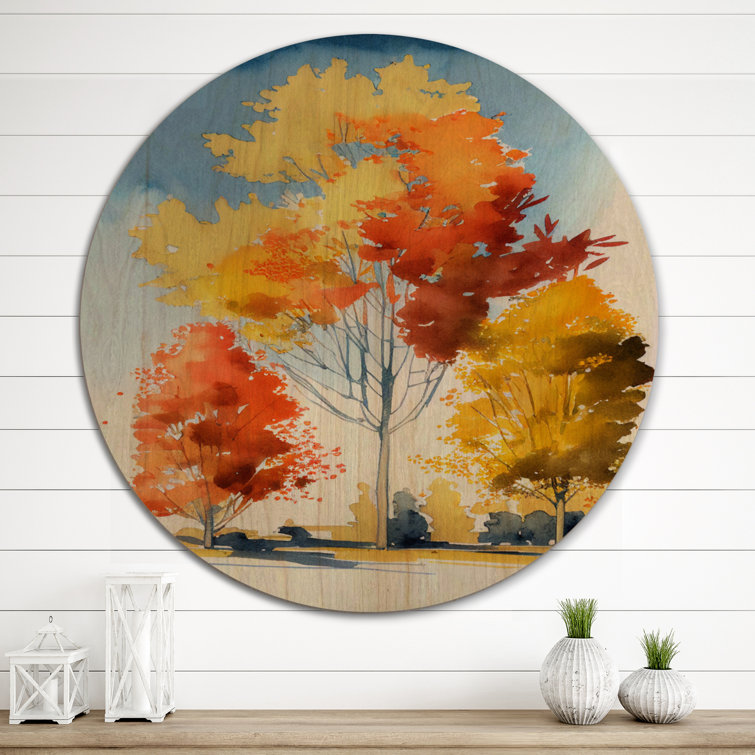The image showcases a circular artistic print mounted on the side of a white house with siding, likely on a deck given the wooden floor visible at the bottom. The art piece, painted on a large circular wooden canvas approximately 4 feet in diameter, vividly depicts an autumn scene with three main trees. The central tree, adorned in a striking combination of red, orange, and yellow leaves, dominates the composition. To its left, a slightly smaller tree displays deep red and orange foliage, while the tree to its right glows with primarily yellow leaves with hints of brown. The sky behind the trees is a serene blend of blue and white. Flanking the artwork at the bottom, there are two white lanterns on the left and two small plants in white pottery on the right. Additionally, two white, face-shaped vases containing tall green grass contribute to the decor, adding an extra layer of visual interest to the serene autumnal display.